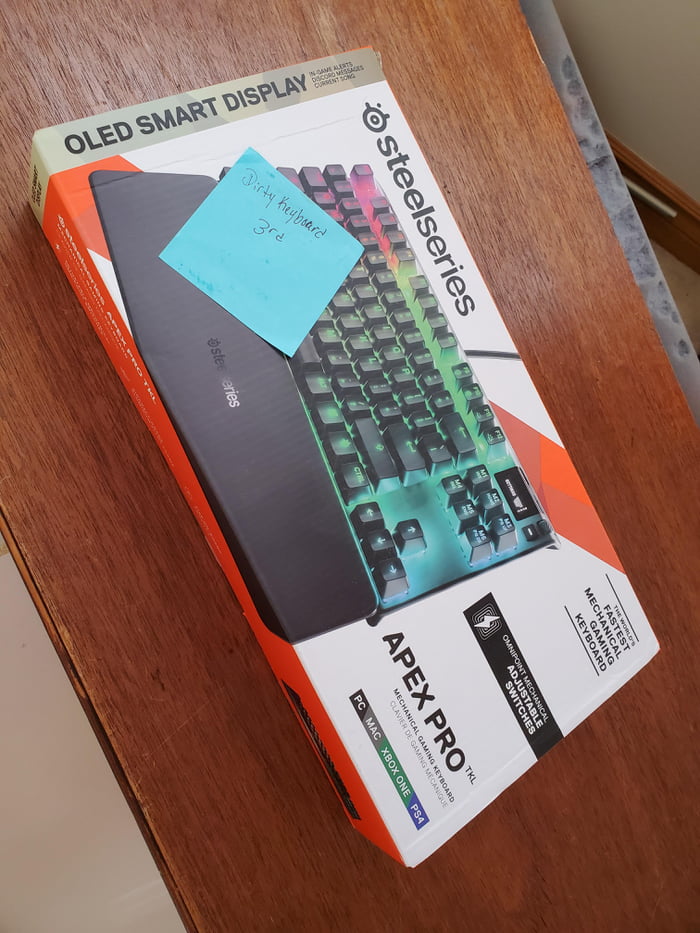A detailed photo showcases a boxed keyboard accompanied by a keyboard wrist pad, placed on a narrow wooden table, reminiscent of a minimalist computer stand. The box features several notable elements: a sticky note with black handwriting affixed at the top left corner, and bold text reading "Apex Pro" at the bottom right corner. Vertical lettering on the left side of the box proclaims "OLED Smart Display," while the brand name "SteelSeries" is displayed at the top left. The tan-colored wall serves as a backdrop, visible both below and at the top right of the box. The photo is currently oriented vertically, but is intended to be viewed horizontally for optimal alignment.